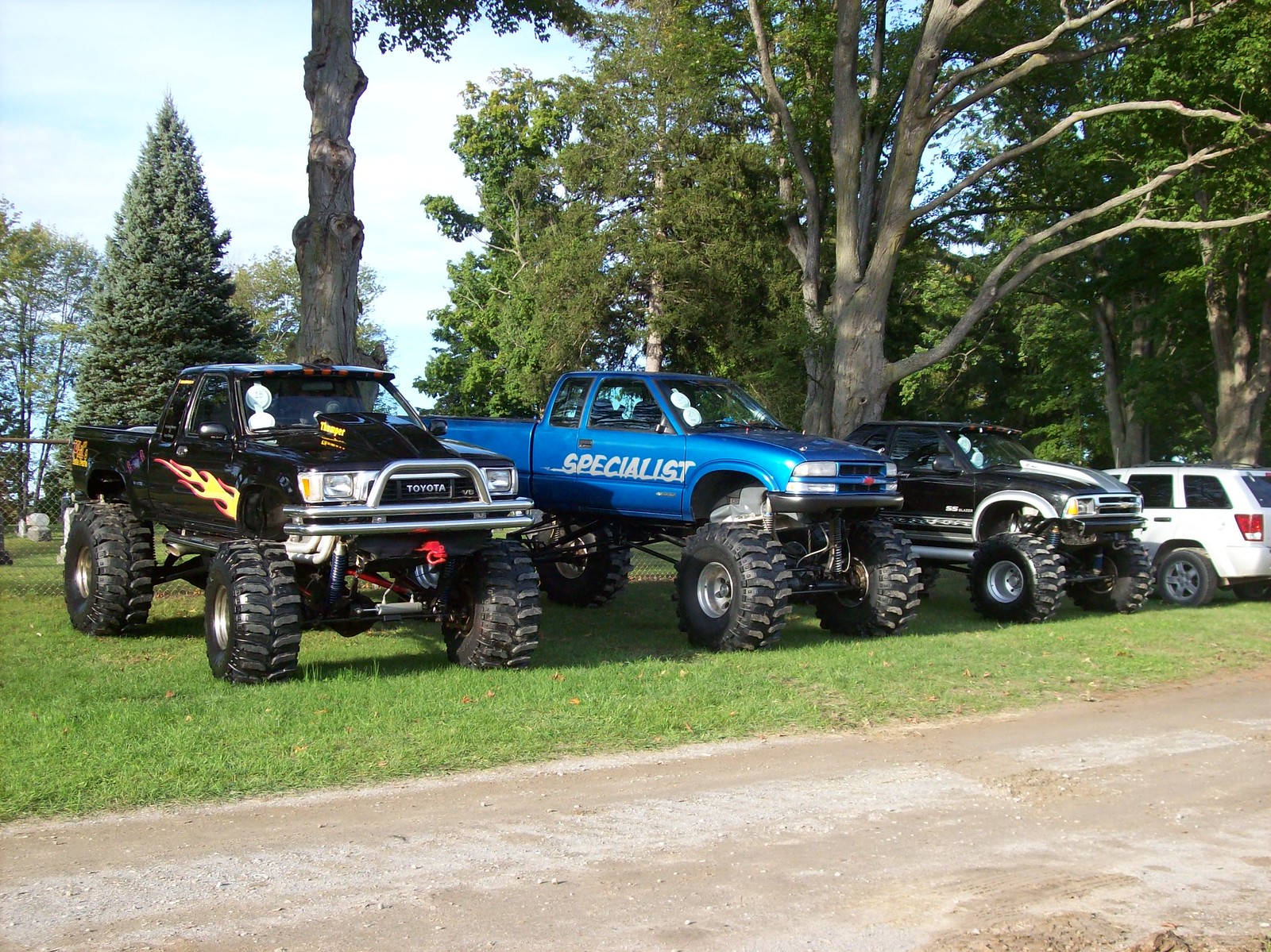This photograph showcases a dynamic lineup of four vehicles parked on a grassy lawn, adjacent to what appears to be either a compacted dirt trail or driveway. Most prominent are three highly modified pickup trucks, each equipped with dramatic lift kits and massive off-road tires that give them the imposing appearance of monster trucks. They are oriented towards the camera at about a 45-degree angle, displaying their formidable right sides.

From left to right, the first truck is a black Toyota pickup adorned with striking red and orange flames along its sides. Following this, a bright blue Chevrolet pickup, labeled 'Specialist', boasts what might be the thickest tires among the trio. Next in line is a smaller black Chevrolet truck, distinguished by a large silver raised hood. The fourth vehicle, a white traditional SUV, is positioned further to the right and faces away from the camera, with part of it cut off from the frame.

Set against a backdrop of several large, leafy trees – including a noticeable cone-shaped deciduous tree and multiple hardwoods – the scene comes to life under a blue sky dotted with light clouds. This compelling arrangement of vehicles, nature, and a hint of urban landscape presents a vivid and detailed portrait of rugged automotive power amidst a serene natural setting.